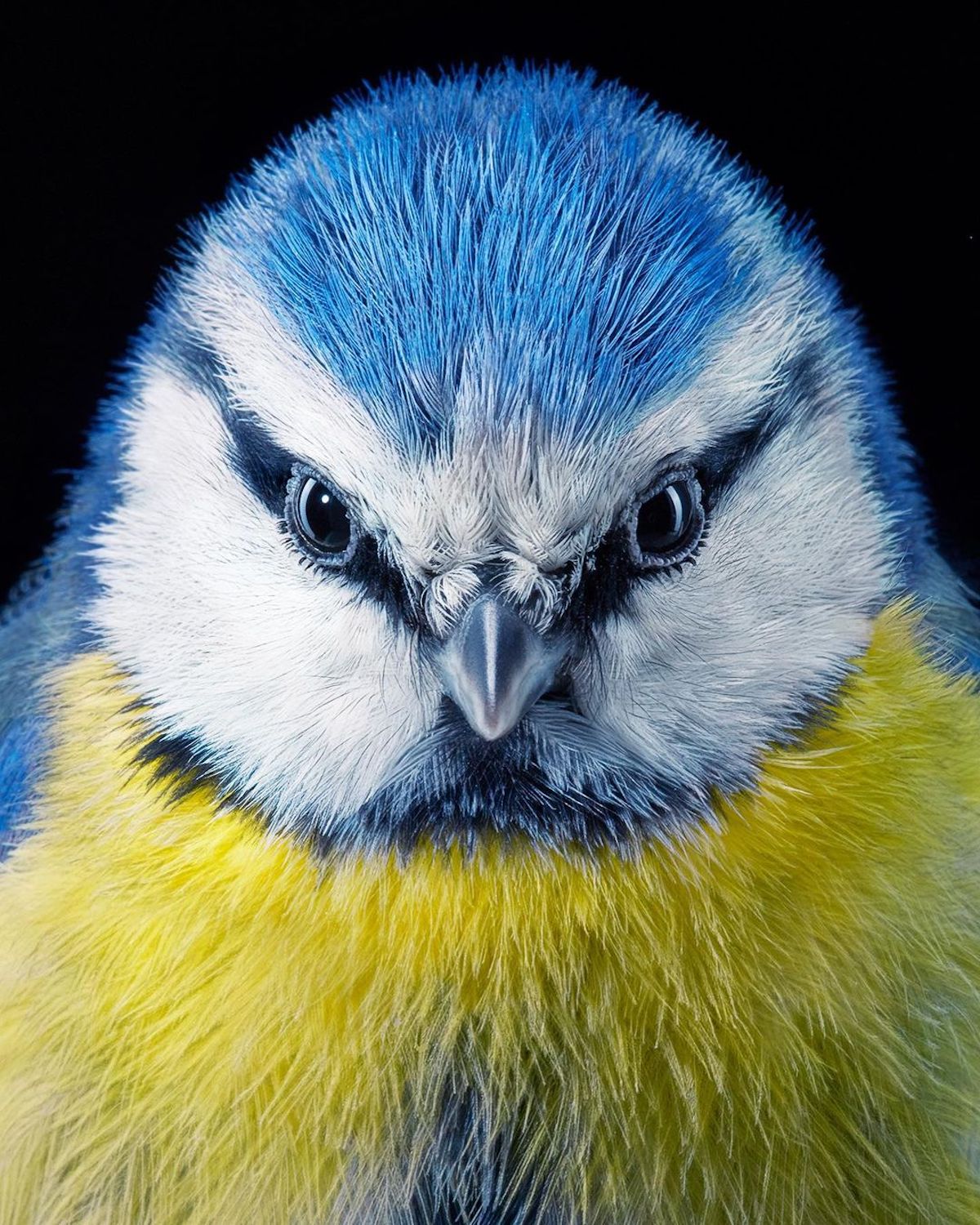The image is a dramatic close-up photograph of a bird's head and neck. The bird's head features a complex pattern of colors: the very top is adorned with blue feathers that extend down the sides, forming a striking line. Beneath the blue, the upper forehead is white, creating a V-shaped pattern. The eyes are dark, bead-like black with a reflective white dot on each, especially noticeable. Thin black stripes run from the beak through the eyes to the sides of the head, giving it a somewhat frowny and intense expression. The beak is sharp, brownish gray, with a distinct white strip on top and a slight plasticky texture. Below the beak, the bird's feathers transition to a white section under the eyes before shifting to a vibrant yellow chest with a subtle blue patch in the center. The background behind the bird is completely black, which accentuates the bird's striking coloration in this close-up shot.